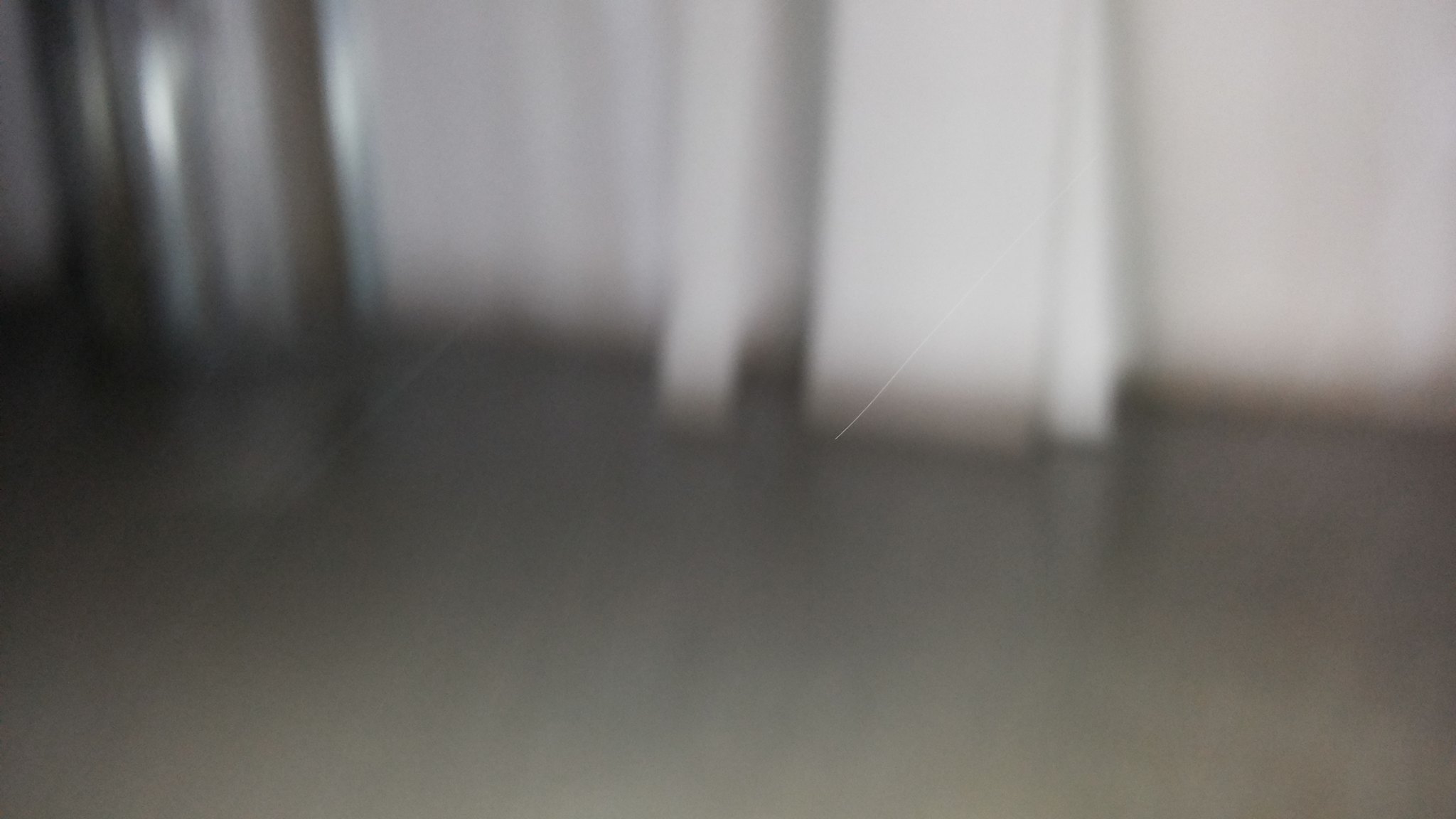The image is a highly blurred rectangular photograph that is approximately 50% wider than it is tall. The bottom half of the image, which seems to depict the floor, transitions from a medium gray at the lower edge to a darker gray toward the middle, suggesting the presence of a light source. The setting appears to be inside a building with what looks like an off-white wall in the background.

At the bottom center of the image, there are three whiteboards of varying widths leaning against the off-white wall. The upper left-hand corner of the image features a reflective silver or steel cylindrical object, possibly a trash can, catching some light. Above this, there is a notable white scratch that diagonally spans from near the middle of the image up toward the left-hand corner.

Additionally, a section of the wall seems to jut out slightly before receding back, forming a rectangular space. This area as well as the general ambiance of the photograph suggests an empty, indoor environment, possibly an unfurnished or under-construction room. The entire photo is marred by scratches, further obfuscating the already indistinct visual details.